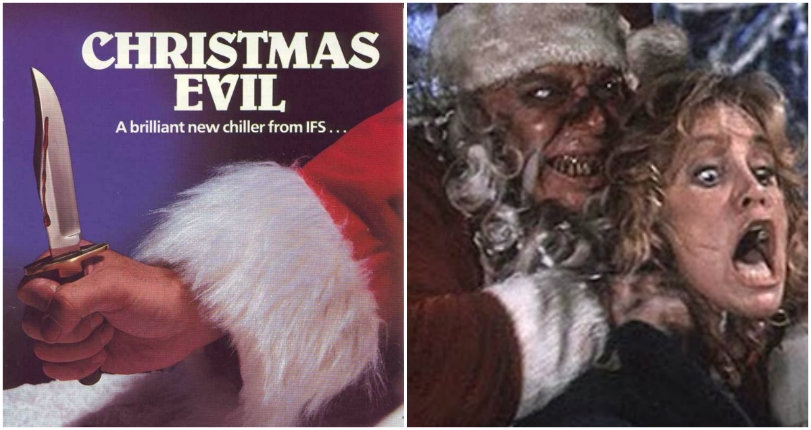The image consists of two distinct but related parts. On the left, it features promotional text in white, stating "Christmas Evil, a brilliant new chiller from IFS." Below this text, an arm clad in a Santa Claus suit emerges, characterized by its red sleeve and white fur trim. The hand holds a blood-streaked knife with a silver blade and gold handle, adding a menacing touch. The background is a mix of blue hues and snowy elements, enhancing the chilling atmosphere.

On the right side, there is a gritty, grainy still from the film, depicting a sinister scene. An evil-looking Santa Claus, complete with a dirty suit, hat, and disheveled beard, is shown. His malevolent eyes and grotesque teeth heighten the horror. He is seen choking a blonde woman, whose mouth is agape in a scream, and her eyes are wide with terror, capturing a moment of intense fear and violence.